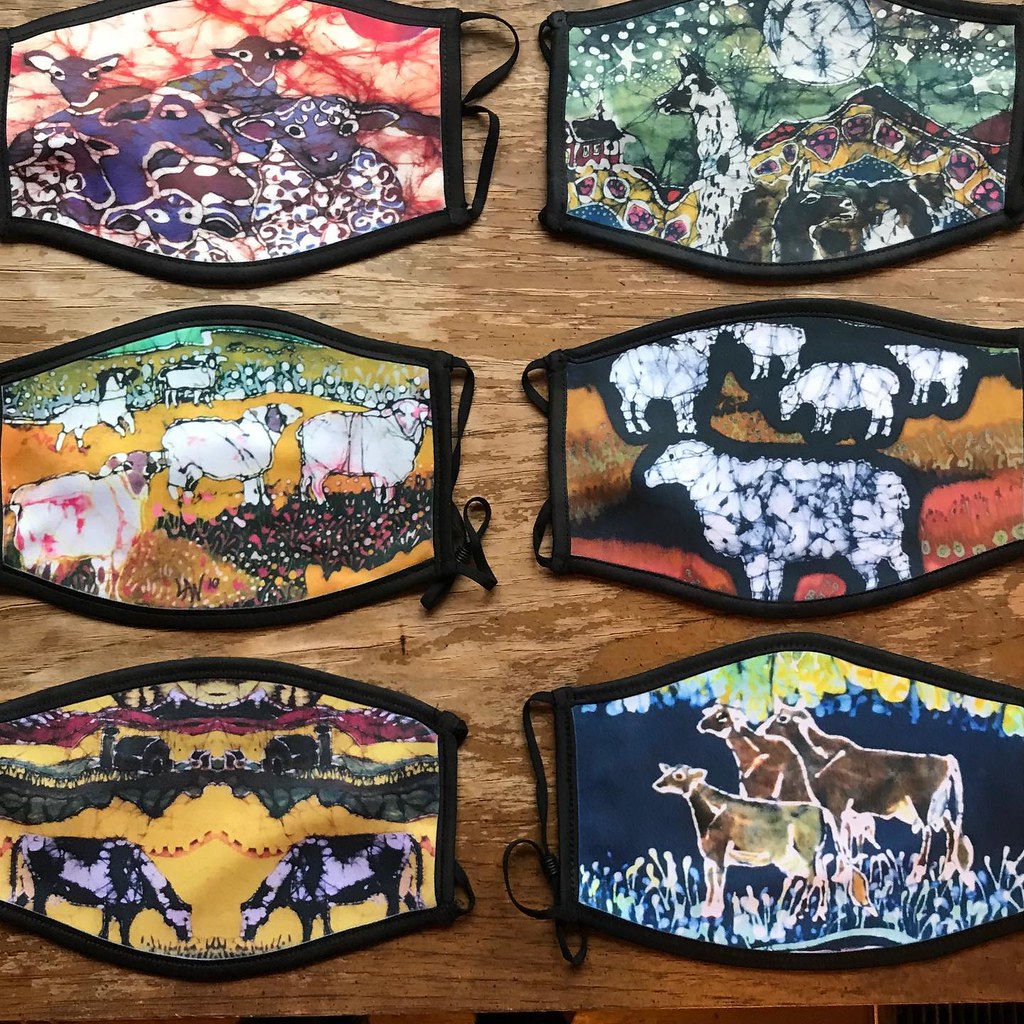In the image, there are six brightly colored face masks adorned with various farm animals, laid out on a rough, faded wooden table that appears to need some finishing. The masks display a vibrant array of colors including yellow, blue, red, orange, magenta, green, black, and white. Starting from the left, the first mask features sheep colored in purple and white with brown spots, set against a peach background with red splotches. The second mask showcases llamas with one having a chocolate brown body and a black head. The background includes colorful mountains, a red house with a black roof, and a green sky with stars and a moon. The third mask depicts sheep with pink spots, grazing on a yellow and orange ground with brown grass and flowers in varying colors, including red and pink. The fourth mask has silhouettes of white sheep with black borders on a landscape transitioning from gold to red. The fifth mask shows black and white cows in a field, flanked by farmhouses, green grass, gold fields, and black and red mountains. The final mask is dark blue with light blue foliage, featuring three chocolate brown deer, with one deer marked with a green patch on its back. All masks are bordered in black and equipped with straps on both sides.